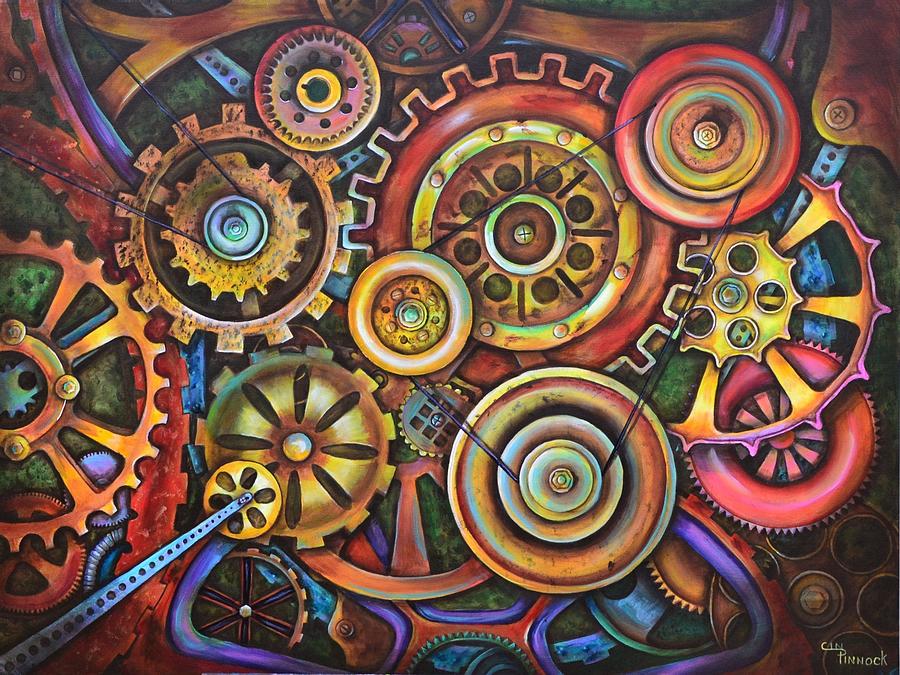The image showcases a highly stylized, colorful painting of interconnected gears, reminiscent of a steampunk aesthetic. The gears, which come in an array of vibrant rainbow iridescent colors including yellowish gold, orange, black, brown, green, blue, magenta, pink, purple, and red, are both large and small. Each gear exhibits unique features; some boast teeth, prongs, and spokes while others are smooth. A network of black pulley strings or belts links these gears, creating an intricate, busy technological composition. The gears appear static and extend from the center towards the edges of the artwork, contributing to an overall surreal and somewhat chaotic visual. Within the detailed scene, there are light blue metal bands and multicolored bolts. An artist's signature is visible at the bottom right, although it is difficult to read. The painting's blend of various elements creates a curious and unrealistic yet captivating piece.